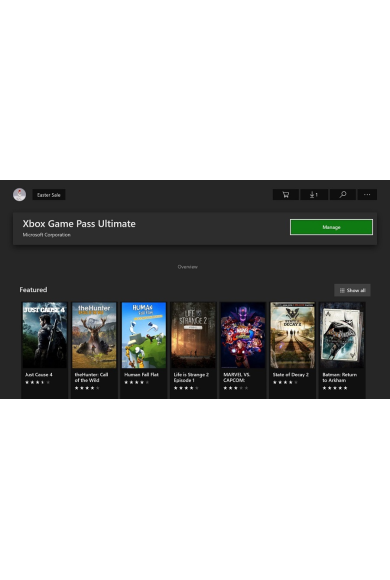The image is a screenshot from a website showcasing the Xbox Game Pass Ultimate. The background of the webpage is predominantly black. At the top of the page, there are multiple utility icons including a shopping cart symbol, a download section, a search area indicated by a magnifying glass, and an options menu represented by three horizontally aligned dots. Directly under the title "Xbox Game Pass Ultimate," the publisher name "Microsoft Corporation" is displayed.

On the right side of the Xbox Game Pass Ultimate title, there's a prominent green button bordered in white with the word "Message" written in white text at its center. Towards the bottom of the screenshot, there is a section titled "Featured," displaying seven different game titles. Each game is presented with its cover image, the title below it, and a star rating indicating its user reviews.